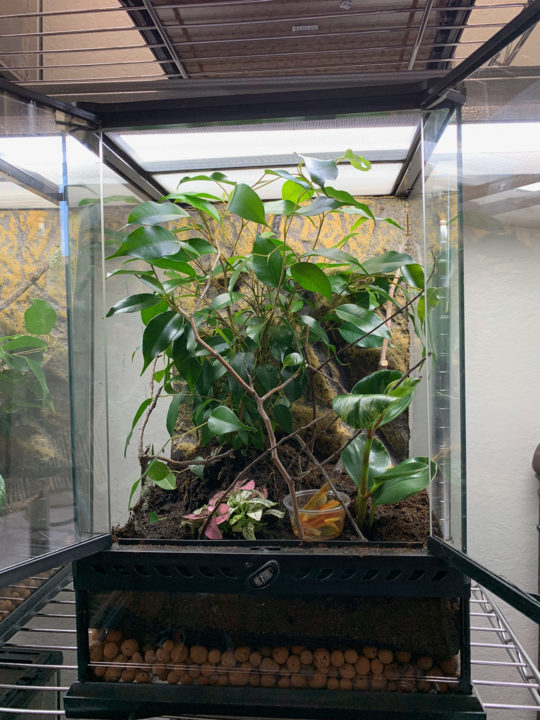This image depicts an indoor terrarium with lush, green foliage. The terrarium, which is a glass enclosure with open doors, showcases a plant with numerous medium-sized, oval leaves that almost seem alive. Inside the terrarium, the plant is anchored in soil resting above a layer of pebbles. A plastic container, presumably a feeding bowl, sits among the foliage, hinting at the possible presence of an unseen animal. The entire setup is situated on a stainless steel grate-like shelf, adding a structural element to the scene. Overhead, a lamp illuminates the terrarium, ensuring the setting is well-lit. The top and bottom edges of the terrarium feature black coloring, framing the verdant interior. Overall, this detailed depiction highlights the vibrant plant life and meticulous setup within the terrarium.